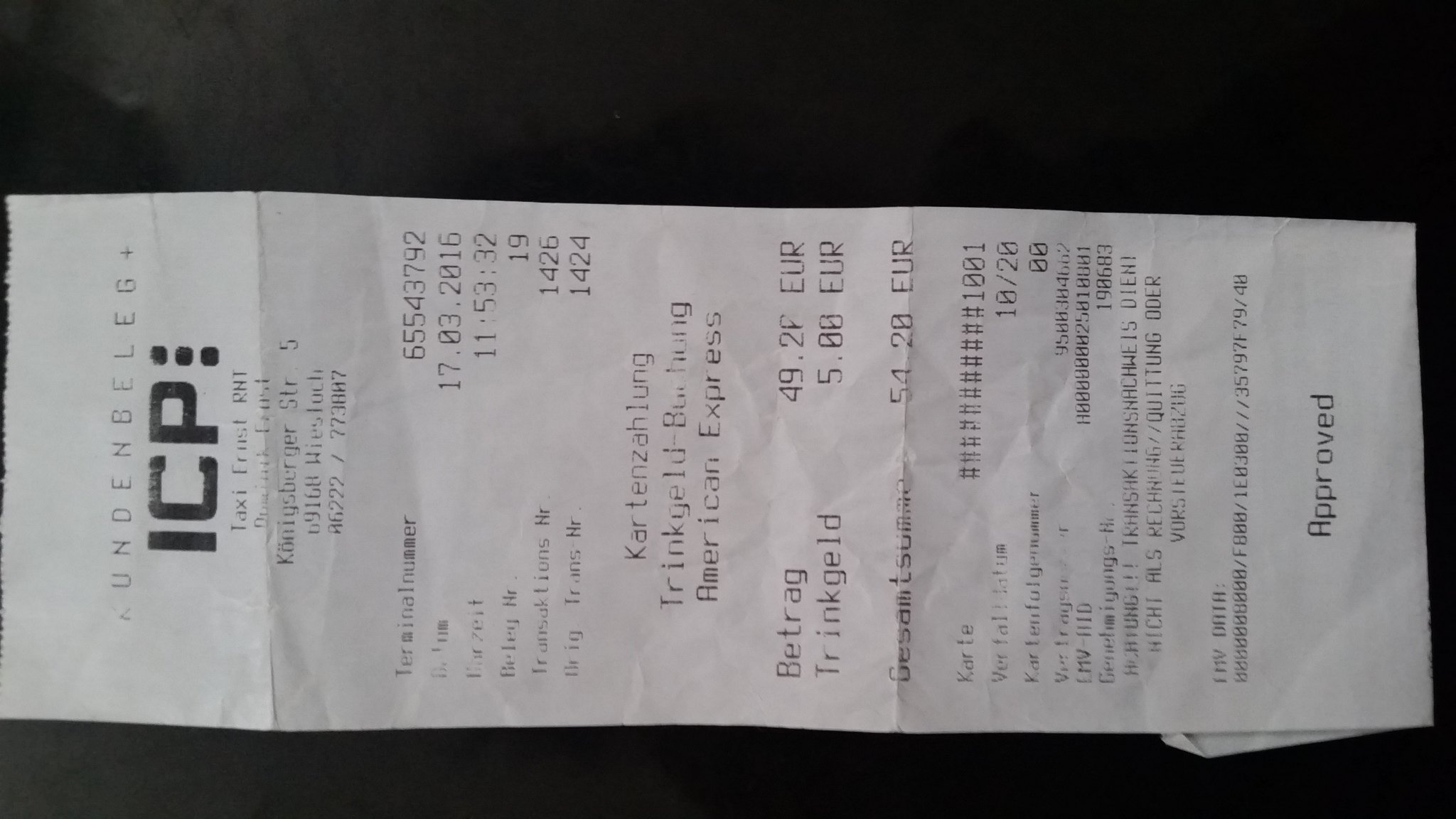This photograph showcases a receipt placed against a black background. The orientation of the receipt is sideways, with the top part positioned on the left side of the image. As a result, the numerical and text elements are vertically aligned rather than horizontally. 

At the top of the receipt, light black lettering is faintly visible. Directly beneath this, the bold, capitalized letters "ICP" are prominently centered. Adjacent to the "P," three solid black rectangles are aligned vertically.

Further to the right, four lines of lighter text detail the receipt's information. Below this section, a list of items purchased is presented, followed by the total amount at the bottom. Centrally at the bottom of the receipt, the word "Approved" is clearly printed, indicating the transaction's completion.